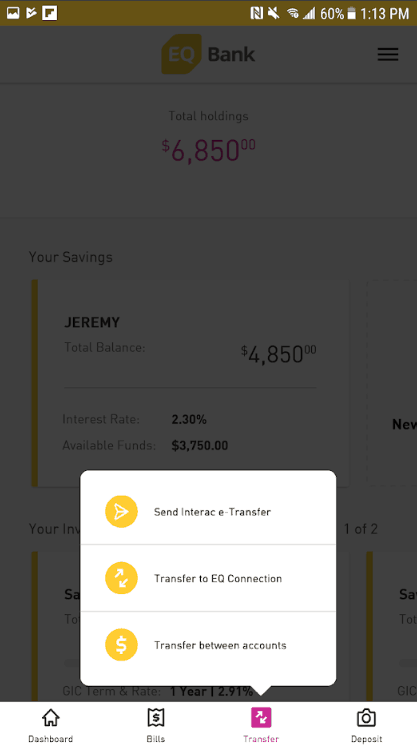Here's a cleaned-up and detailed caption for the given image:

---

The screenshot appears to have a grayscale gradient at the top, transitioning to a brown and gold mixture below. On the upper left-hand side, there are several symbols enclosed within a square with a white border: a white mountain icon, an overturned triangle with a check mark inside, another square with a thick white border depicting stairs, and a notification symbol. Close to these icons, a speaker icon with a line through it signifies that the phone is muted. Nearby, there’s a Wi-Fi symbol with a shield, followed by a full cellphone signal indicator, a battery icon showing 60% charge, and the time displayed as 1:13 PM.

Below this section, within a gray silhouetted area, there's a yellow 3D box marked with bold white text reading "EQ". Adjacent to this, in black text, is the phrase "This Bank", followed by three horizontal lines. Beneath these lines, in the center, it says "Total Holdings" in black, followed by "$6,850" in red text.

On the left-hand side, there's a partial view of a face in a new rectangle. Next to this rectangle, in black text, it says "Your Savings". Below this, two rectangles are positioned together with a yellow and gold band across the top, labeled "JEREMY" in bold black text. Underneath, in dark gray text, it states "Total Balance" and to the right in black text, "$4,850." Another gray rectangle below this indicates the "Interest Rate" at "2.3%" in black text, and further down it lists "Available Funds" at "$3,750" in gray text.

A pop-up rectangle appears white with gray line separations, dividing it into three smaller rectangles. Each smaller rectangle contains a gold circle with different images inside. These act as clickable areas, including a hot pink square with directional arrows and the label "Transfer" in hot pink lettering beneath it. Above this, a chat bubble with a triangle pointer indicates interaction.

The three options within the pop-up are:
1. A white butterfly icon with the label "Send INTERAC e-Transfer" in black text to the right.
2. An icon with arrows pointing up and down, labeled "Transfer to EQ Connection".
3. An "S" symbol with lines at the top and bottom, labeled "Transfer between Accounts".

At the bottom bezel on the left-hand side, there’s a black silhouette of a house with the label "Dashboard" underneath. Adjacent is a wavy ribbon icon with a dollar sign, labeled "Bills". Following this is the "Transfer" option, and finally, a camera body silhouette with a circle in it, marked "Deposit".